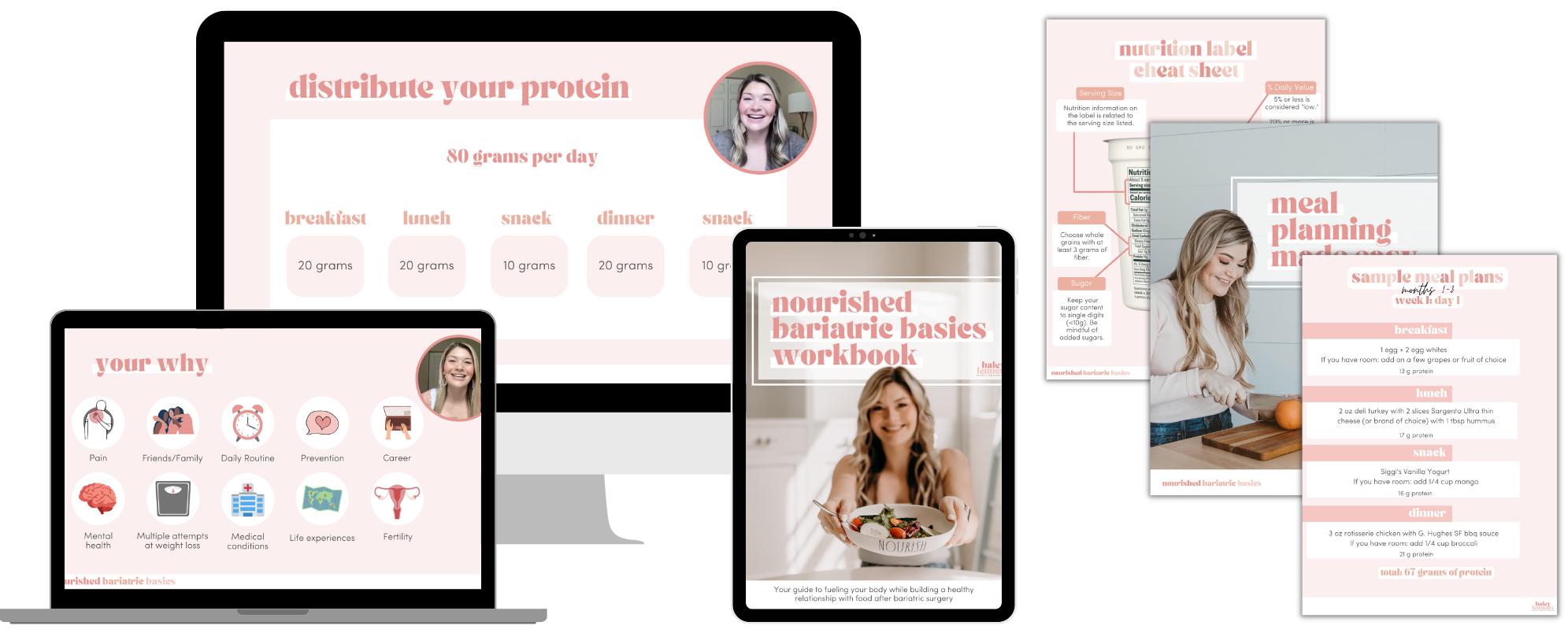On a clutter-free workspace, a sleek black desktop monitor with a white base displays a detailed nutrition plan with pink and black text. The screen reads "Your Protein: 80 grams per day" in pink, followed by an itemized list in black specifying "Breakfast 20 grams, Lunch 20 grams, Snack 10 grams, Snack 10 grams, Dinner 20 grams." To the left, a laptop positioned in the corner focuses on motivational factors, entitled "Your Why," in plain black text. Key motivators are highlighted, like "Pain, Friends, Family, Daily Routine, Prevention, Career, Mental Health, Multiple Attempts at Weight Loss, Medical Conditions, Life Experiences, Fertility." 

Situated in the right corner, a matching black tablet showcases the "Nourish Bariatric Basics Workbook" in pink. The screen features an image of a woman holding a white bowl of salad, with the term "Nourish" bolded in black. Below it, black text explains, "A guide to fueling your body while building a healthy relationship with food after bariatric surgery." Three stacked pages appear beneath the title, each annotated in pink and black. The bottom page is titled "Nutrition Label Cheat Sheet," the middle "Meal Planning Made Easy," and the top "Sample Meal Plans." The sample meal plan section includes a timeline: "Months 1 to 3," and specifies a detailed plan for "Week 1... Day 1," breaking down meals into categories: "Breakfast, Lunch, Snack, and Dinner."